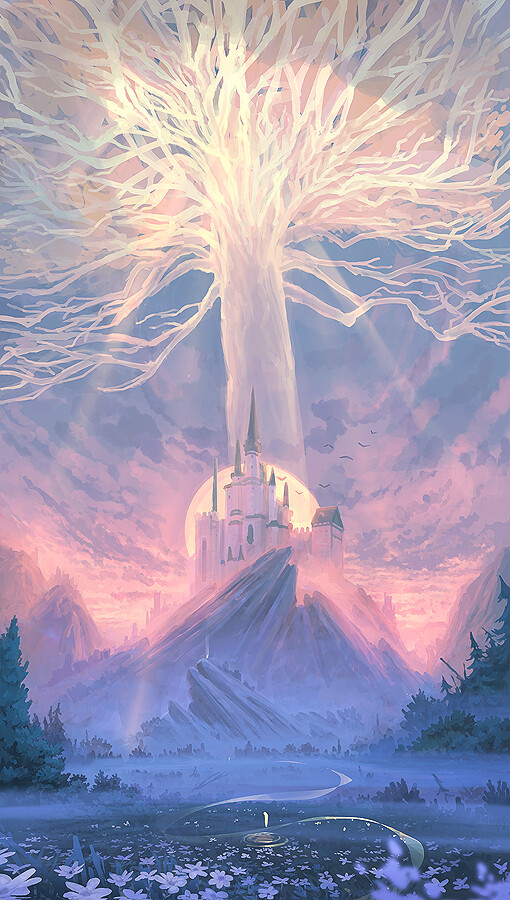In the forefront of the artwork lies a serene field blanketed with delicate white flowers, creating a calm and inviting scene. This floral expanse gently fades into a dense, forested area on either side, characterized by stately evergreen trees that contribute to the depth and complexity of the piece. Beyond these trees, the terrain rises dramatically into sharp, jagged mountains that carve a majestic silhouette into the distant skyline. Perched upon these formidable peaks stands a magnificent castle, its white walls and greenish-gray rooftops imbued with an ethereal glow. The castle's architecture features numerous slender, needle-like spires that ascend gracefully towards the heavens. Dominating the upper region of the image, a mystical tree composed entirely of light emerges, radiating an otherworldly brilliance. This luminous tree, mostly bare of leaves, showcases an intricate network of glowing branches and a resplendent trunk, emanating rays of light that cascade downwards, illuminating the entire scene in a magical ambiance. The sun, positioned behind the castle, casts a divine halo around the entire composition, enhancing the dreamlike quality of this captivating landscape.